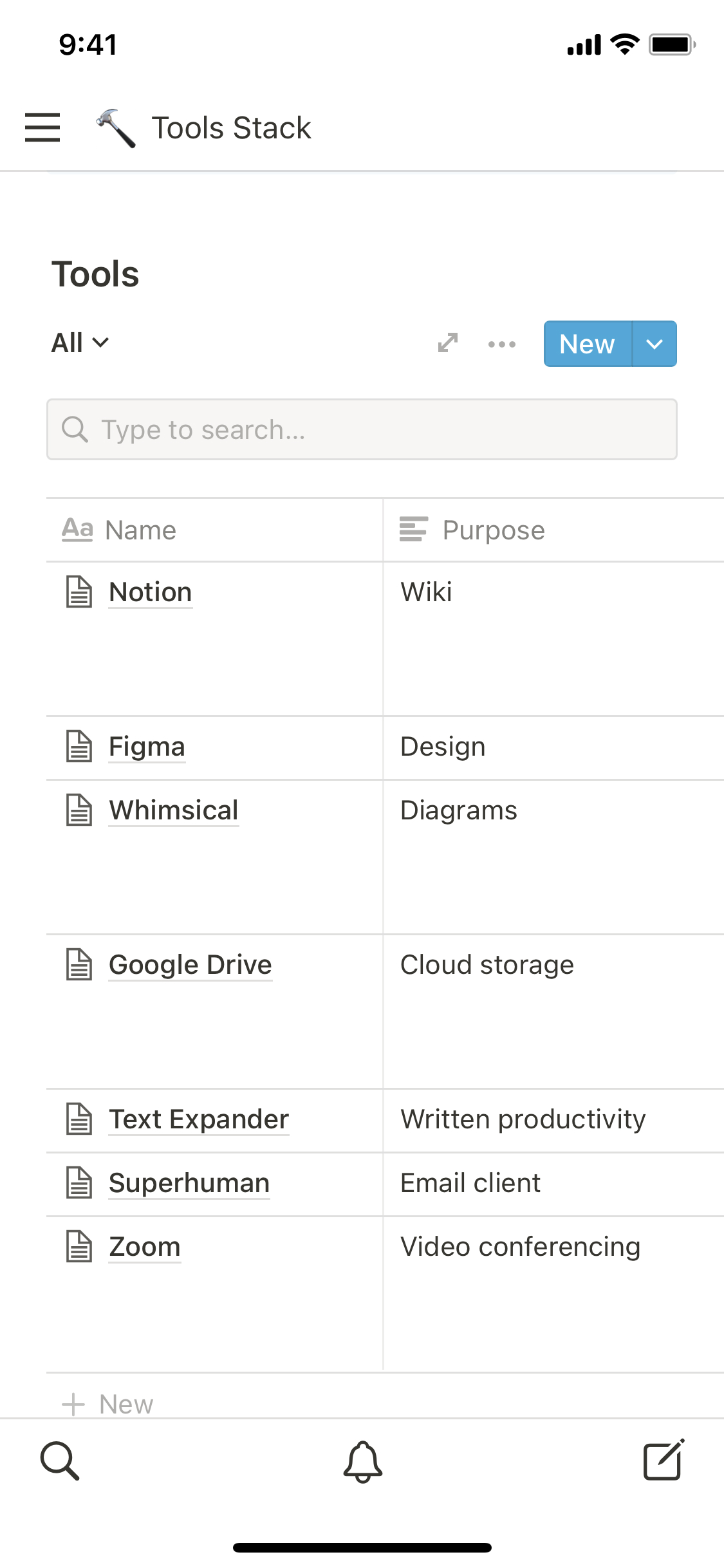The image features a user interface on a white background. At the top left corner, the time is displayed as "9:41." Below the time, there is an icon with three horizontal lines next to a hammer symbol, labeled "Tool Stack." Directly beneath this, there is a dropdown box labeled "Tools" with a downward arrow beside it. 

Adjacent to this dropdown, there is an icon with an up-and-down arrow and three vertical dots. To the right, there is a blue button labeled "New" with a downward arrow beside it, followed by a blue search bar.

Below this section is a box with large and small underlined "A" symbols, labeled "Name." Underneath are items listed: "Notion," "Figma," and "Whimsical." Subsequently, there are individual boxes labeled: "Google Drive," "TextExpander," "Superhuman," and "Zoom."

On the right side, there's a small note icon with lines titled "Purpose." Below this are more boxes labeled: "Wiki, Design and Diagrams," "Cloud Storage," "Written Productivity," "Email Client," and "Video Conferencing." 

At the bottom of the interface, there is a long box labeled "+ New." To the far bottom, there are icons of a magnifying glass, a bell, a square with a pencil, and a long black dividing line.